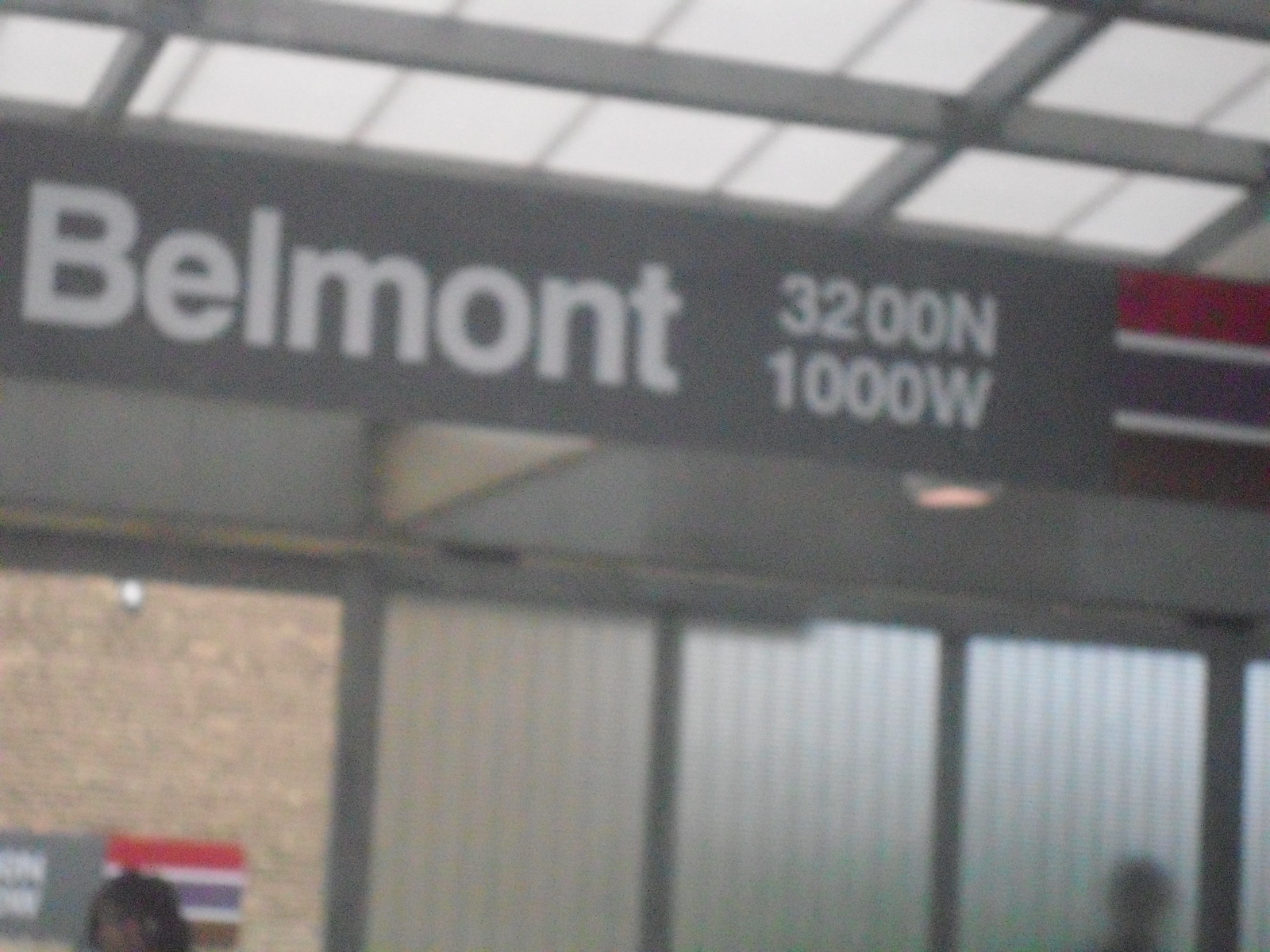This image appears to be taken at a bus or train station, likely in Chicago, as indicated by the "Belmont" sign accompanied by "3200 North, 1000 West" in large white letters on a gray strip. The scene is set in a semi-enclosed outdoor space under a skylight bordered in black, allowing light to shine through the translucent panels. The background includes beige brick sections with window panels bordered in dark gray and lighter in the middle, possibly casting silhouettes of people behind them. In front of the brick structure, there's a notable sign with red, gray, and brown stripes, alongside a gray box and the silhouette of a person with black hair and a brown face. A red and white banner also features prominently in the image. The overall composition, including the granulated quality, suggests this could be an older photo or one taken in a public transit setting.